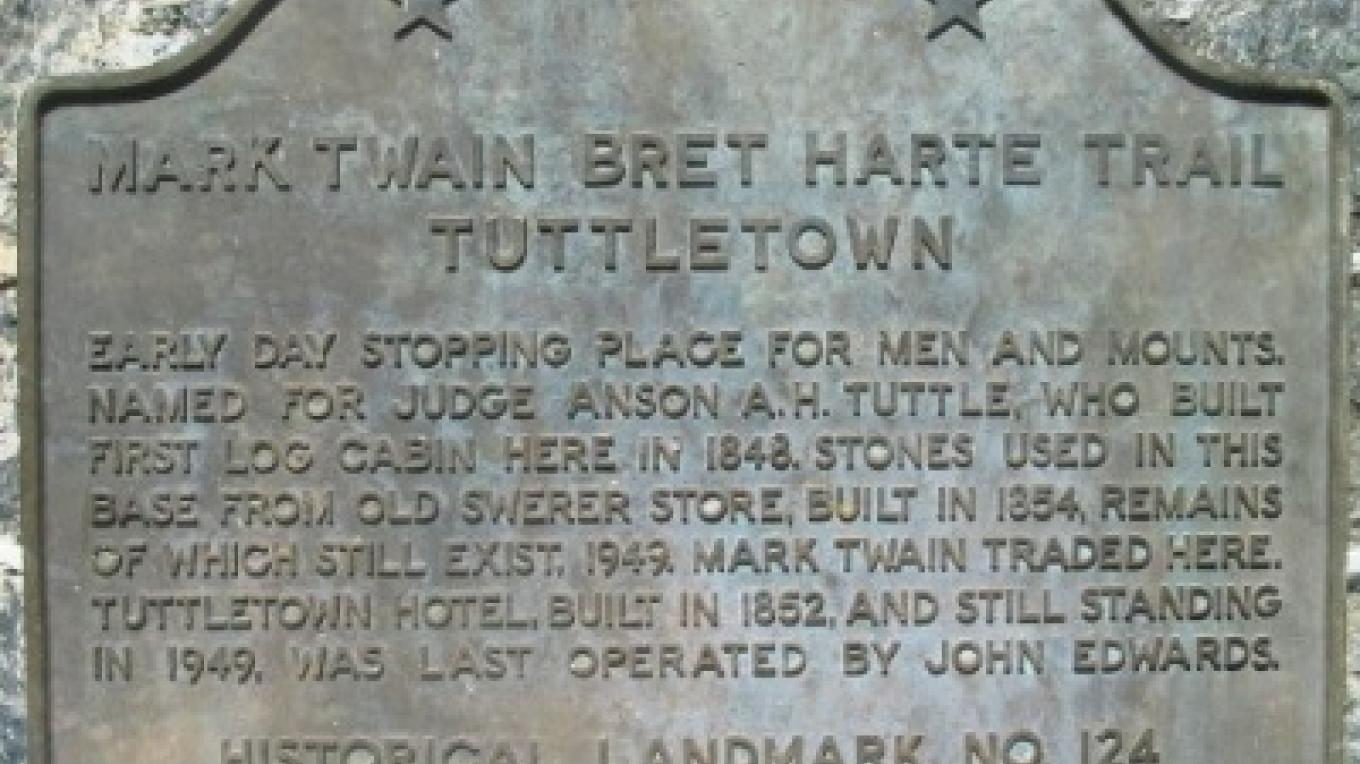This black-and-white photograph captures a weathered grey historical marker, set in what appears to be a cement or metal surface with a patina. The marker, rectangular but cropped at the top and bottom in the image, has two stars at its pinnacle. The raised lettering on the marker reads: "Mark Twain Bret Hart Trail, Tuttletown." Below, in smaller but still prominent raised text, it details an early stopping place for men and their mounts, named after Judge Anson A. H. Tuttle, who built the first log cabin here in 1848. The inscription continues, stating that the stones used in the base are from Old Swearer's Store, built in 1858, with remains still existing in 1949. It also mentions that Mark Twain traded here. Additional information includes that the Tuttletown Hotel, built in 1858 and still standing in 1949, was last operated by John Edwards. The bottom portion of the marker, partially cut off in the photograph, labels it as Historical Landmark Number 124, inscribed as "Historical Landmark N.O. 124."